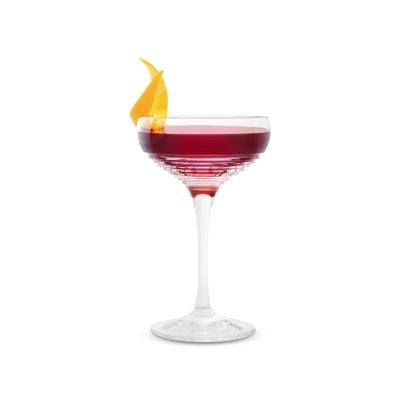The image showcases a striking, single object centered against a completely white background: a clear glass with a long, thin stem and a wide opening. The glass contains a light red to maroon liquid that nearly reaches the top. Notably, an orange garnish or peel is visibly hanging on the left side of the rim, while an unusual flame or fiery embellishment seems to emerge from the same area. Additionally, the liquid inside the glass exhibits potential horizontal white lines or reflections. The overall composition is minimalistic, carrying a clean and somewhat promotional aesthetic, making it suitable for use on social media or possibly as a digital image for a drink advertisement. The colors featured prominently are white, yellow, orange, maroon, and clear.